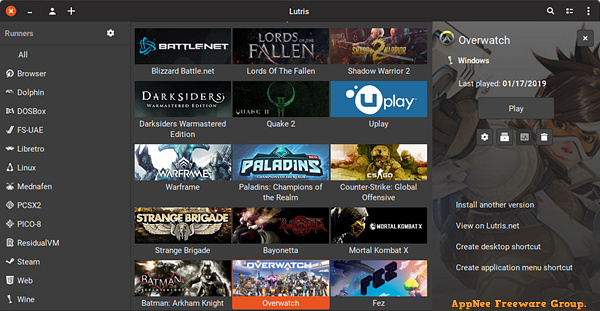The image shows a detailed interface of a game application or game store. The categories and platforms listed include Browser, Dolphin, DOSBox, FS-UAE, Libretro, Linux, MedNothing, PCSX2, PICO-8, Residual VM, Steam, Web, and Wine. The games showcased within this interface feature popular titles such as Battlenet, Darksiders, Warhammer, Warframe, Strange Brigade, Paladins: Champions of the Realm, Counter-Strike: Global Offensive, Overwatch, Mortal Kombat X, and Bayonetta. The layout is clean and organized, indicating a well-structured platform designed to cater to a wide variety of gaming preferences and interests.